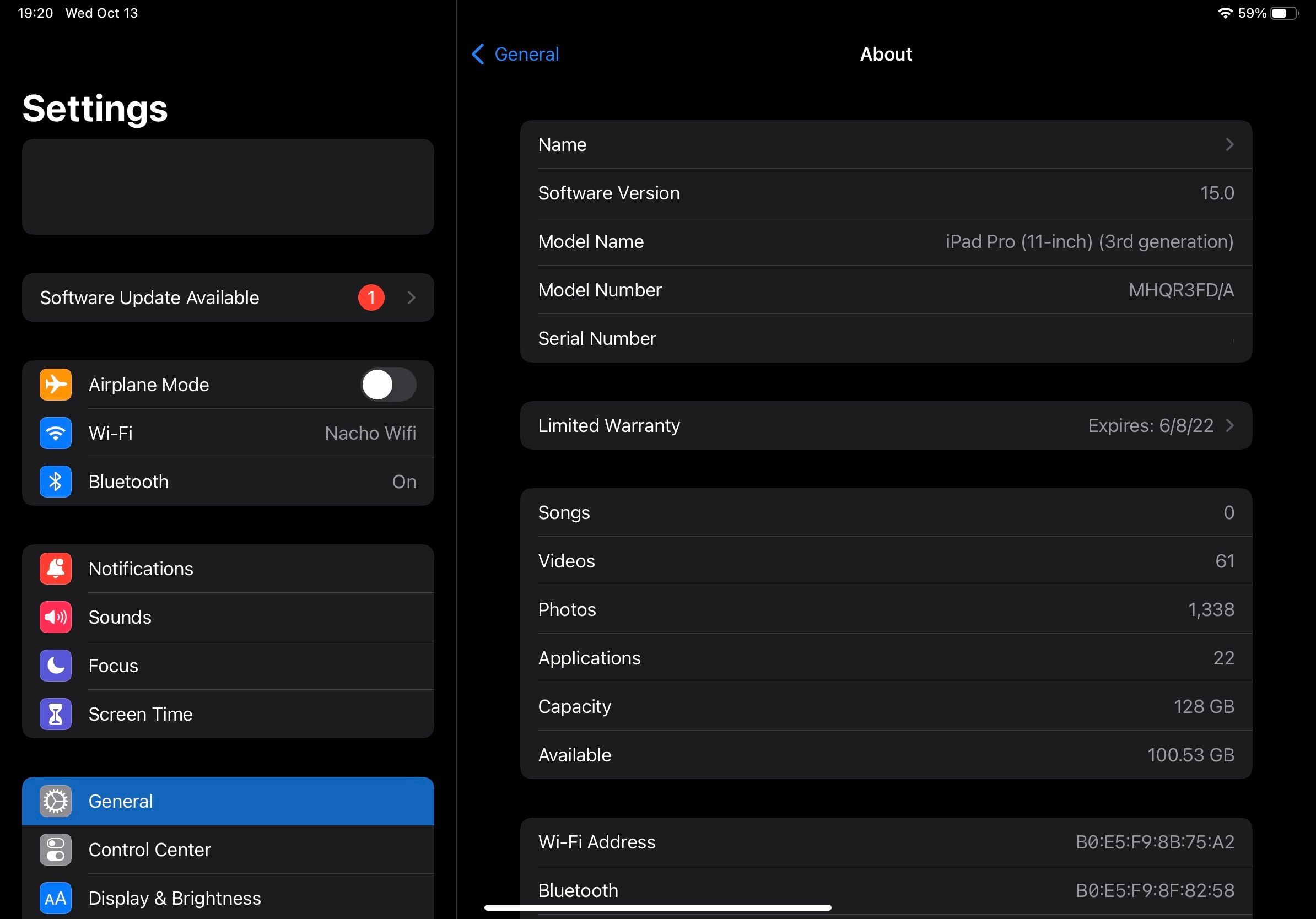This screenshot depicts the settings screen of a device in dark mode, set against a black background. In the upper left-hand corner, the white text denotes the time as 19:20, along with the day, WED (Wednesday), and the date, OCT 13. On the far right of the page, the signal strength is represented by five bars, and the battery indicator shows 59% with a half-full battery icon next to it.

Central to the image, a blue back arrow pointing to the left appears alongside the blue text "General." To the right of this, the word "About" is displayed in white. Below this, “Settings” is written on the left, followed by an empty, slightly lighter black box. Below this box is another similar box which is thinner and contains the text "Software update available," highlighted by a red circle with a white number "1" inside it.

Further down, the screen features various icons and settings options. At the top left of this section, a yellow box with a white airplane signifies "Airplane Mode," with a toggle switch indicating that airplane mode is off (right circle pulled to the left). Beneath it, a blue box with a white Wi-Fi icon indicates the Wi-Fi connection status with the network named "NachoWi-Fi."

The next box contains a blue icon with the Bluetooth symbol, indicating Bluetooth connectivity status alongside the text "Bluetooth" and the word "On." Directly underneath, a red box with a white bell denotes "Notifications," followed by another red box with a white horn icon labeled "Sounds." All text is in white. 

Subsequently, a purple box features a white crescent moon icon labeled "Focus," and below that is another purple box with an hourglass icon labeled "Screen Time." Further down, a section starts with a gray box containing a white gear icon alongside the text "General." Underneath, a gray box with two white symbols represents the control center accessibility, labeled "Control Center."

To the right of the label "General," a blue box with two white 'A's indicates "Display Brightness." Another section details the device information, including "Software Version," which shows "15.0," and "Model Name" labeled "iPad Pro (11-inch) (3rd generation)." Below, the "Model Number" reads "MHQR3FDJA," and "Serial Number" with associated details.

Next, under "Limited Warranty," it states "Expires: 6-8-22." There are separate boxes listing media information: "Songs" with a count of zero, "Videos" at 61, "Photos" at 1,338, and "Applications" at 22. The device's "Capacity" is displayed as "128 GB," with "Available" space of "100.53 GB." Finally, the "Wi-Fi Address" is given as "B0:E5:F9:H8:75:A2," and the "Bluetooth" address is "B0:E5:49:8F:82:58."